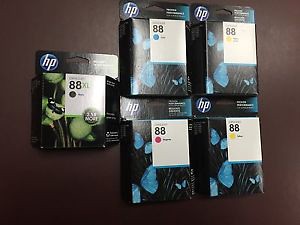The image depicts five Hewlett-Packard (HP) printer ink cartridges arranged on a brown surface. Each cartridge is marked with the numbers "88XL" or "88" to signify compatibility with specific HP printers. Four of the boxes have a predominantly black background adorned with turquoise blue imagery resembling blobs. The fifth box, which seems to be an extra-large cartridge, stands out with its green and black design. Additionally, each package contains small colored dots for identification: red, yellow, yellow, blue, and a black dot on the green cartridge. The packaging also features a distinct hanging lip labeled with "HP," although the exact product details are not explicitly clear from the image alone.